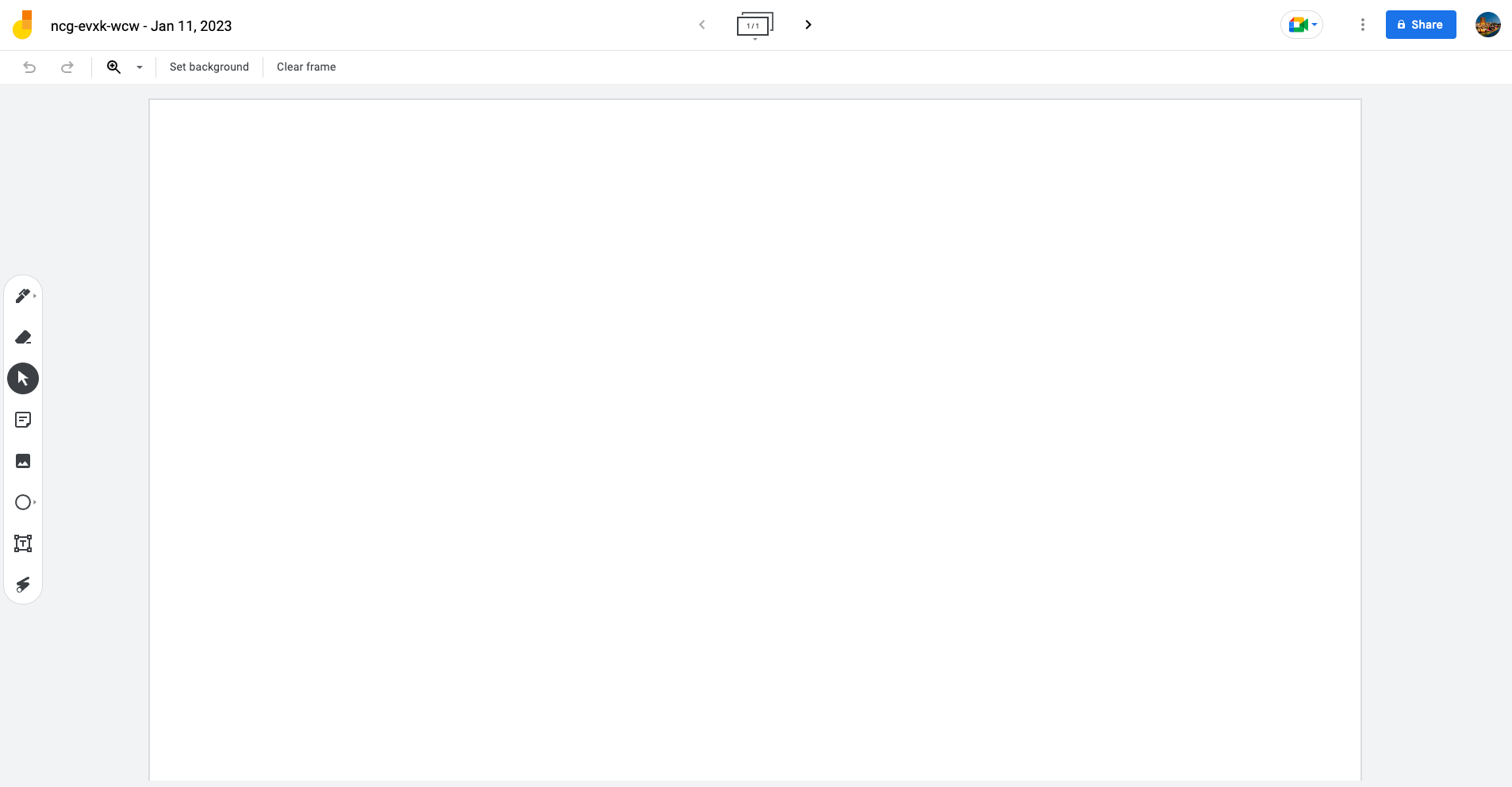The image features a variety of symbols and shapes, arranged in a complex layout:

1. A yellow circle containing an orange bar positioned at the top, accompanied by some text and a date.
2. To its left, an arrow points to the left.
3. Nearby, a filled rectangle appears with another rectangle beneath it, along with a rightward-pointing arrow.
4. On the right side, there's a symbol comprised of green and yellow colors, with vertical dots stacked on top of each other.
5. Further right, a blue rectangle contains a symbol and a word inside it, followed by a circle with an embedded picture.
6. Moving back to the left, there is a gray area followed by a magnifying glass and additional text that isn't completely legible.
7. Below this section, a gray rectangle frames a white rectangle, which is empty.
8. Within the gray rectangle on the left, several indistinct symbols can be observed:
   - The first or second symbol is not clear.
   - The third symbol depicts a black circle with a white arrow pointing towards the upper left.
   - Another unclear symbol follows.
   - A black square.
   - A gray outlined circle.
   - An additional ambiguous symbol.
   - A final, indiscernible shape.

Overall, the image comprises various geometric shapes and colored symbols interspersed with text, creating a somewhat intricate visual composition.